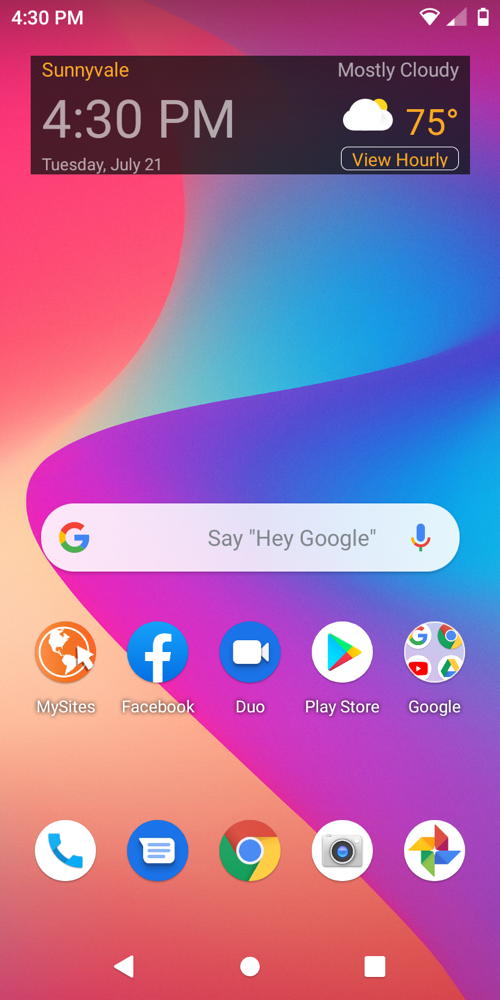The image appears to be a screenshot of a smartphone's home screen, featuring a vibrant background with a gradient of colors. In the upper left corner, a hot pink hue transitions to a light blue in the upper right. As we move downward, the light blue darkens into a deeper blue, which then fades into a purple hue toward the bottom right. The left side of the screen displays an orange color.

At the top of the image, within a black box, the word "Sunnyvale" is highlighted in orange. To the right of this, it indicates that the weather is "mostly cloudy." Below this text is a graphic showing a cloud with the sun behind it, next to the temperature reading of 75 degrees, with an option to "view hourly" forecasts underneath. To the left of the cloud icon, the time is displayed as 4:30 p.m., and below that, in smaller text, is the date: Tuesday, July 21st.

Approximately four inches down from the top, there is a Google search bar with the prompt "Say 'Hey Google'" accompanied by a microphone icon. The next row features quick access to several apps: My Sites, Facebook, Duo, Play Store, and Google. 

Continuing down to the bottom row, there are several icons: a white circle with a blue phone inside, a blue circle with a white notebook inside, the Google Chrome icon, a white circle with a camera inside, and a white circle with the Google logo colors (red, green, yellow, blue) arranged in different directions.